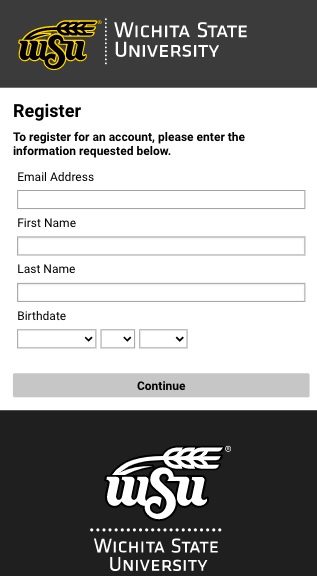Captured from a cell phone, this image features a screen displaying the Wichita State University registration page. At the top, framed in a light to dark grayish rectangle, is the text "Wichita State University" alongside an emblem depicting a curling grain of wheat with the letters "WSU" beside it, where the 'S' stands prominently larger. 

The middle section is predominantly white, hosting the registration form. It begins with the word "Register" followed by a message: "To register for an account, please enter the information requested below." 

The form fields include boxes labeled “Email Address,” “First Name,” and “Last Name.” Below these fields are dropdown menus for birth date selection, formatted to request the year first, followed by the day and month.

At the bottom of the form is a long, slim, gray rectangle button labeled "Continue" in black letters. Below this, toward the lower part of the image, there is a larger black rectangle containing the wheat emblem and "WSU" letters. Beneath a dotted line, it once more reads "Wichita State University."